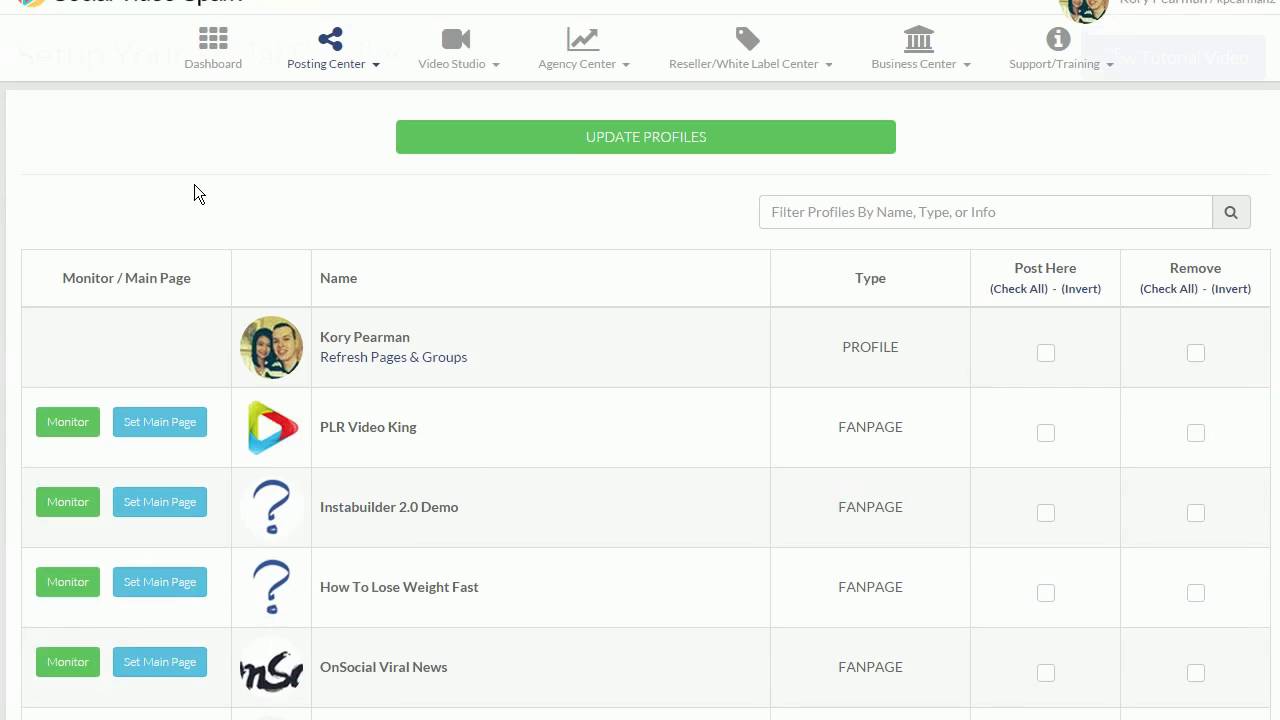This image captures the interface of a digital device screen, partially obscured at the top, cutting off the company's name. The background is primarily white, with faint gray lines creating subtle separations into distinct sections. At the top of the screen, a navigation menu is visible, listing options like "Dashboard," "Posting Center," "Video Studio," "Agency Center," "Reseller/White Label Center," "Business Center," and "Support Training."

Below this menu, a prominent green button labeled "Update Profiles" is centrally located in the upper section of the screen. On the right side, there is a search bar with the placeholder text "Filter profiles by name, type, or info." The layout is organized into columns, with headings such as "Monitor/Main Page," icons or pictures beneath each heading, "Name," "Type," "Post Here," and action options like "Check All," "Invert," "Remove."

Specifically under the "Monitor/Main Page" section, there are green buttons labeled "Monitor" and "Set Main Page," with four instances of each. Additionally, recognizable Disney symbols are seen within the "Google Play" area. This detailed interface appears to be part of a management or administrative tool, designed for handling various digital profiles and tasks efficiently.